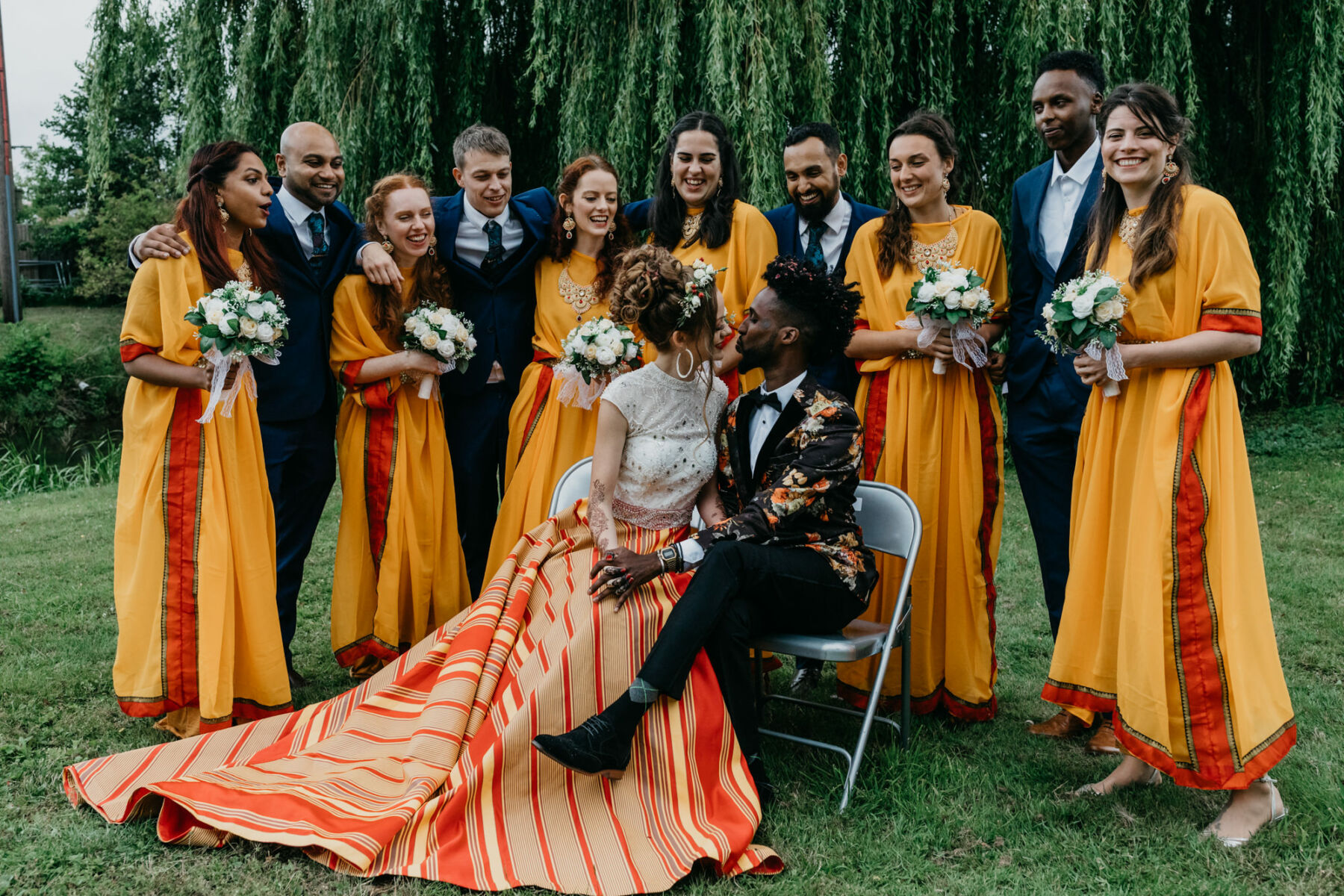In this vibrant outdoor wedding scene, the bride and groom sit close together on two metal chairs, one blue and one white, front and center in the photo. They're about to kiss, their faces inches apart, holding hands and exuding a palpable sense of affection. The groom, an African American man with dreads and a short beard, is dressed in a stylish navy blue suit paired with black pants and suit shoes. The bride, adorned in a flowing white dress, has floral tattoos on her arm and is gazing intently at her groom. She holds a bouquet of white flowers, which is a common detail among all the bridesmaids. Behind them, the backdrop features a giant tree with dangling greenery and a lush grass lawn. The bridal party consists of ten individuals, all beaming with joy and focusing on the happy couple. The men are uniformly dressed in navy blue suits, while the women wear traditional orangish-red patterned dresses with red armbands. The groomsmen and bridesmaids stand side by side, alternating, with their hands affectionately placed over each other's shoulders, creating a cohesive and joyous group.